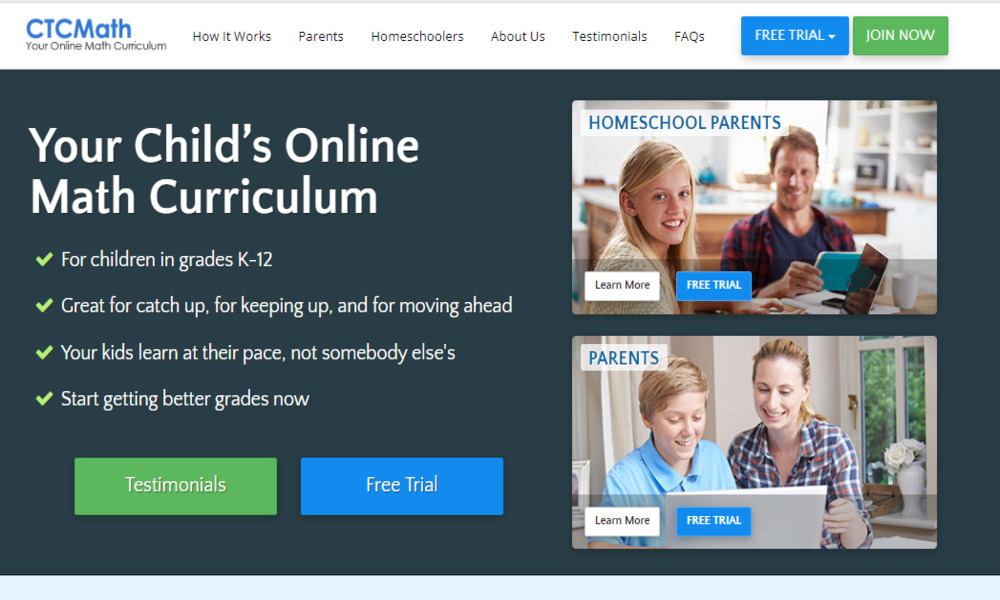This image is a screenshot from a website featuring an online math curriculum. The main background of the site is dark grey, contrasting with a white navigation bar at the top. In the top left corner of the navigation bar, the text "CAPITALS CTCMATH" is displayed in blue, followed by a small "ATH". Below this, a tagline reads, "Your online math curriculum." 

On the top right of the navigation bar, there is a series of navigation options: "How it works," "Parents," "Homeschoolers," "About us," "Testimonials," and "FAQs." Further to the right, a blue button with white text says "FREE TRIAL" and features a drop-down menu. Adjacent to this is a green button with white text reading "JOIN NOW."

In the dark grey section of the site, large white text on the left announces, "Your child's online math curriculum." Listed below are four bullet points, each emphasized with a green tick mark:

1. For children in grades K to 12.
2. Great for catch up, keeping up, and moving ahead.
3. Your kids learn at their pace, not somebody else's.
4. Start getting better grades now.

Centered beneath these bullet points are two buttons: a green one labeled "Testimonials" and a blue one labeled "FREE TRIAL," both in white text.

On the right side of the website, two landscape-oriented photographs are displayed. The first photo features a young girl smiling at the camera, with her father slightly out of focus beside her. The top left corner of this image contains the text "Homeschool Parents," along with buttons for "Learn More" and "Free Trial." 

Below this, the second photo depicts a mother and child looking at a laptop. The top left corner of this image is labeled "Parents," also accompanied by buttons for "Learn More" and "Free Trial."